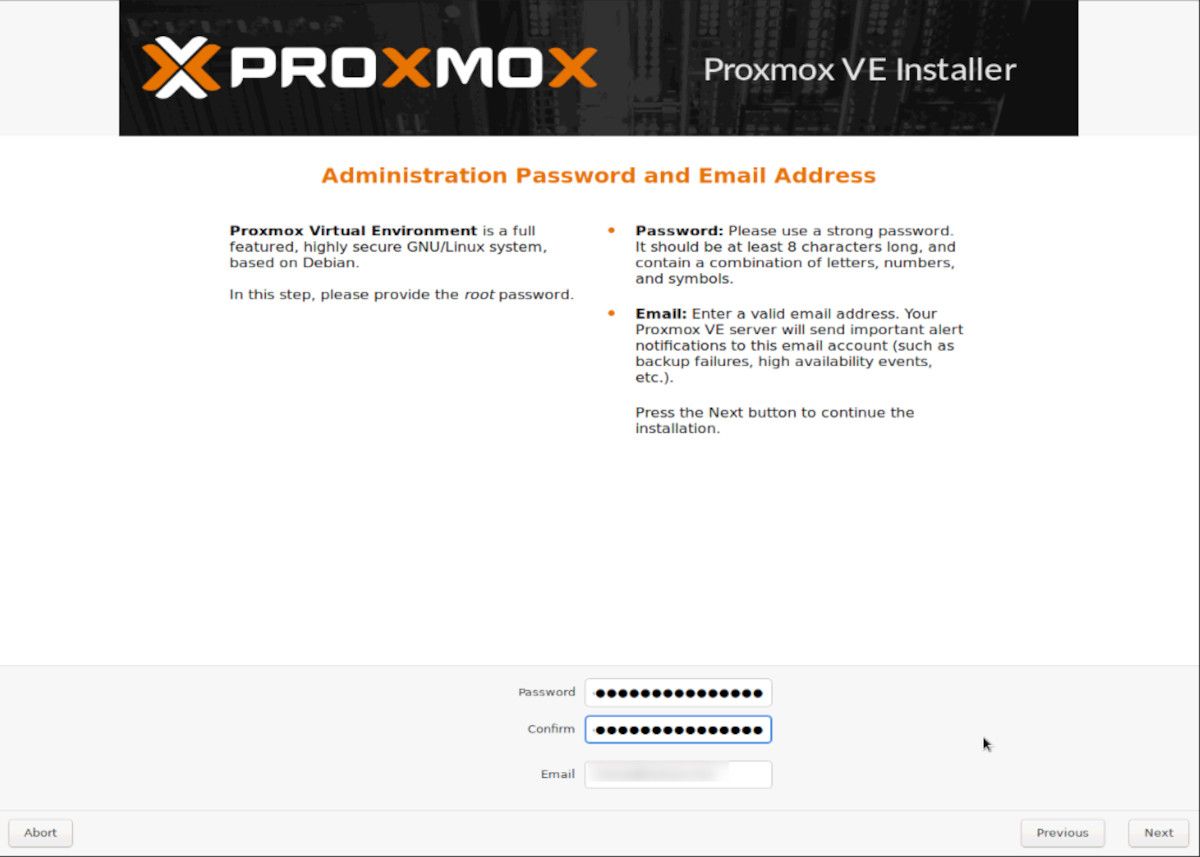The screenshot depicts a section from a webpage featuring a predominantly white background with a dark gray header. The header, characterized by a textured pattern of vertical lines in varying shades of gray, prominently displays the "PROXMOX" brand name. The lettering of "PROXMOX" is styled distinctively with "PRO" in white, followed by an orange "X", "MO" in white, and finishing with an orange "X". Accompanying the text is a logo consisting of four triangles, arranged to form an "X" shape, utilizing both the white and orange color scheme. 

On the right end of the header, white text reads "PROXMOX VE installer." Directly below this, against a white background, the orange text "Administration password and email address" is displayed. Below this heading, a brief explanation in gray provides further details. Further down, a light gray footer features input fields for a password and its confirmation, obscured by black dots, and an email address field, which has been grayed out for privacy.